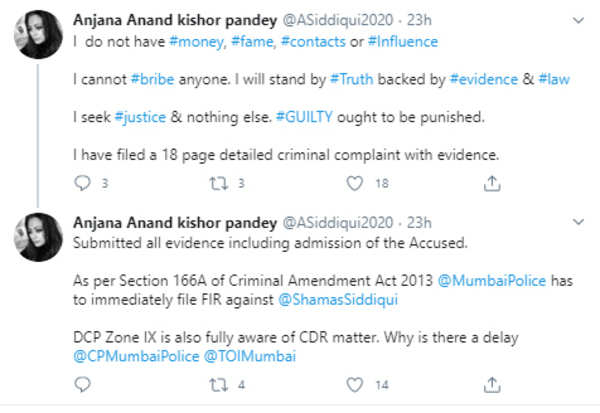Here's a cleaned-up and detailed caption for the image described:

---

This image is a screenshot of two consecutive tweets from the same user, @asadiki2020, whose real name is Anjana Anand Kishore Pandey. The profile picture in the tweet shows a black and white photo of a woman wearing a headscarf, holding a cell phone, and taking a selfie. Her face is turned to her right.

Posted 23 hours before the screenshot was taken, the first tweet reads:

"I do not have #money, #fame, #contacts, or #influence. I cannot #bribe anyone. I will stand by #truth backed by #evidence and #law. I seek #justice and nothing else. #Guilty ought to be punished. I have filed an 18-page detailed criminal complaint with evidence."

This tweet has received 3 comments, 3 retweets, and 18 likes.

The text of the second tweet continues directly from the first:

"Submitted all evidence including the admission of the accused. As per section 166A of Criminal Amendments Act of 2013, Mumbai Police has to immediately file an FIR against @ShamaSiddiqui. DCP Zone 9 is also fully aware of the CDR matter. Why is there a delay, @CPMumbaiPolice @TOIMumbai?"

The second tweet has garnered 4 retweets and 14 likes but no comments.